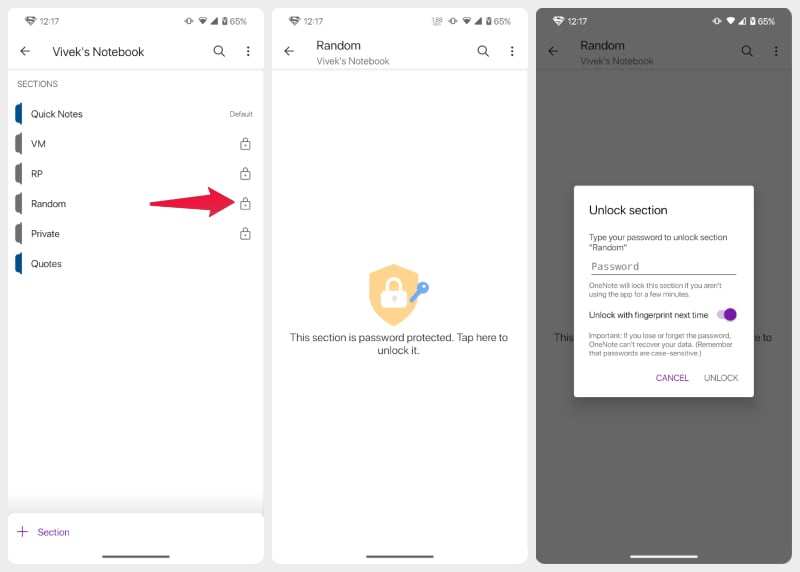The image contains three sequential screenshots of a digital note application, all showcasing a phone with a Superman logo in front of the time reading "12:17" and a battery level at 65%. 

1. The first screenshot displays "Vivek's Notebook," with sections labeled "Quick Notes," "VM," "RP," "Random," "Private," and "Quotes." There is an arrow pointing from "Random" on the left side to the right side.

2. The second screenshot focuses on the "Random" section of Vivek's Notebook. This section is indicated to be password protected, featuring an image of a key and a lock. It includes a note saying, "This section is password protected. Tap here to unlock it."

3. The third screenshot shows the unlocked process of the "Random" section in Vivek's Notebook. It prompts the user to "Type your password to unlock section 'Random'." A password input field is available, with a note below stating, "OneNote will lock this section if you aren't using the app for a few minutes."

These screenshots visually narrate the process of navigating through a protected section within Vivek's digital notebook.